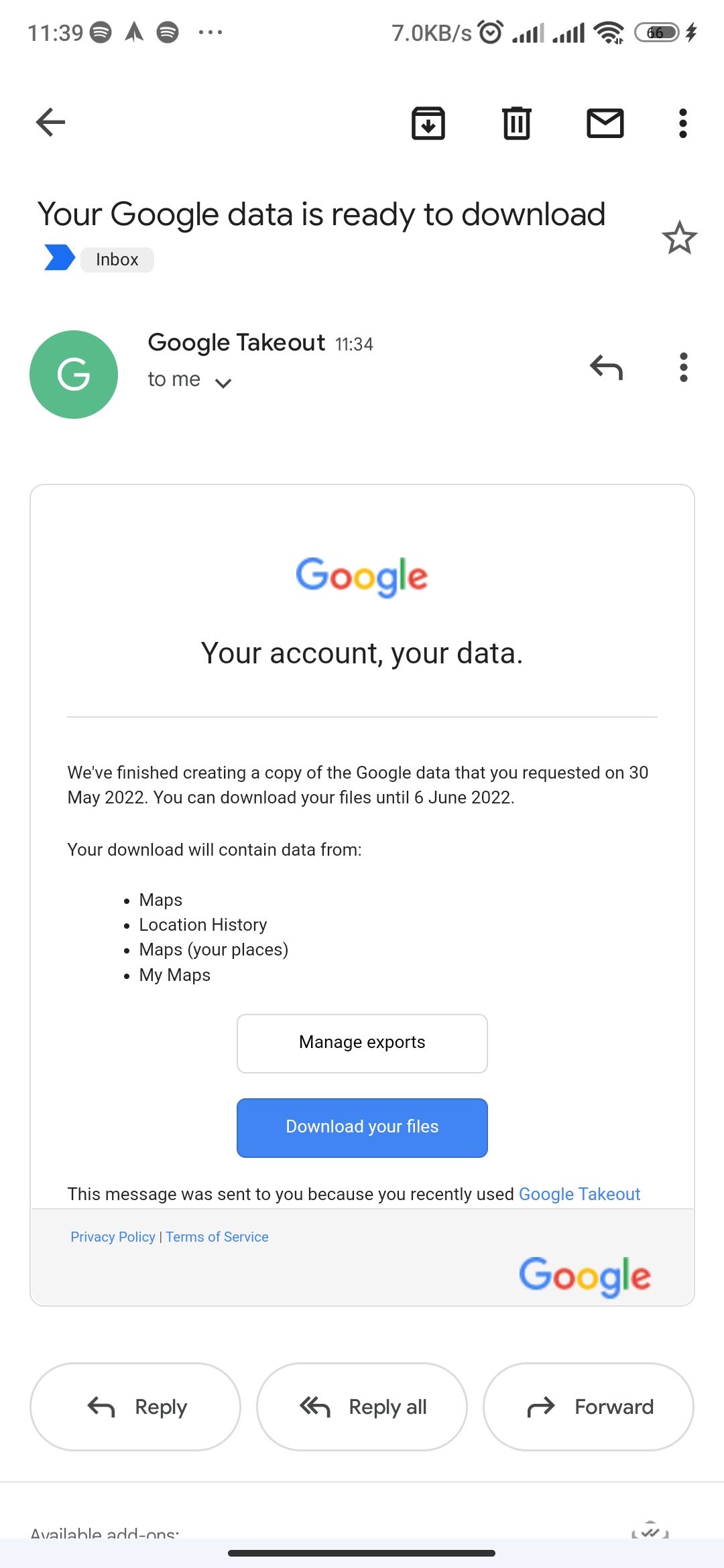This image is a screenshot of a notification email from Google. At the top, a message in bold declares, "Your Google Data is ready to download." Below this, a green circle highlights the Google Takeout logo next to the time "1:34." Just underneath, there is a dropdown arrow labeled "to me." The Google logo, in its signature colorful style (blue G, red o, yellow o, blue g, green l, red e), is prominently displayed below this.

The main body of the email reads: "Your account, your data. We finished creating a copy of the Google data that you requested on 30 May 2022. You can download your files until 6 June 2022. Your download will contain data from:
- Maps
- Location History
- Maps (your places)
- My Maps"

Following this, two buttons are visible. The first button, in white with black text, says "Manage exports." The second button, in blue with yellow text, indicates "Download your files."

At the bottom of the email, it states in black text, "This message was sent to you because you recently used Google Takeout." Finally, there are links to the Privacy Policy, Terms of Service, and Google.